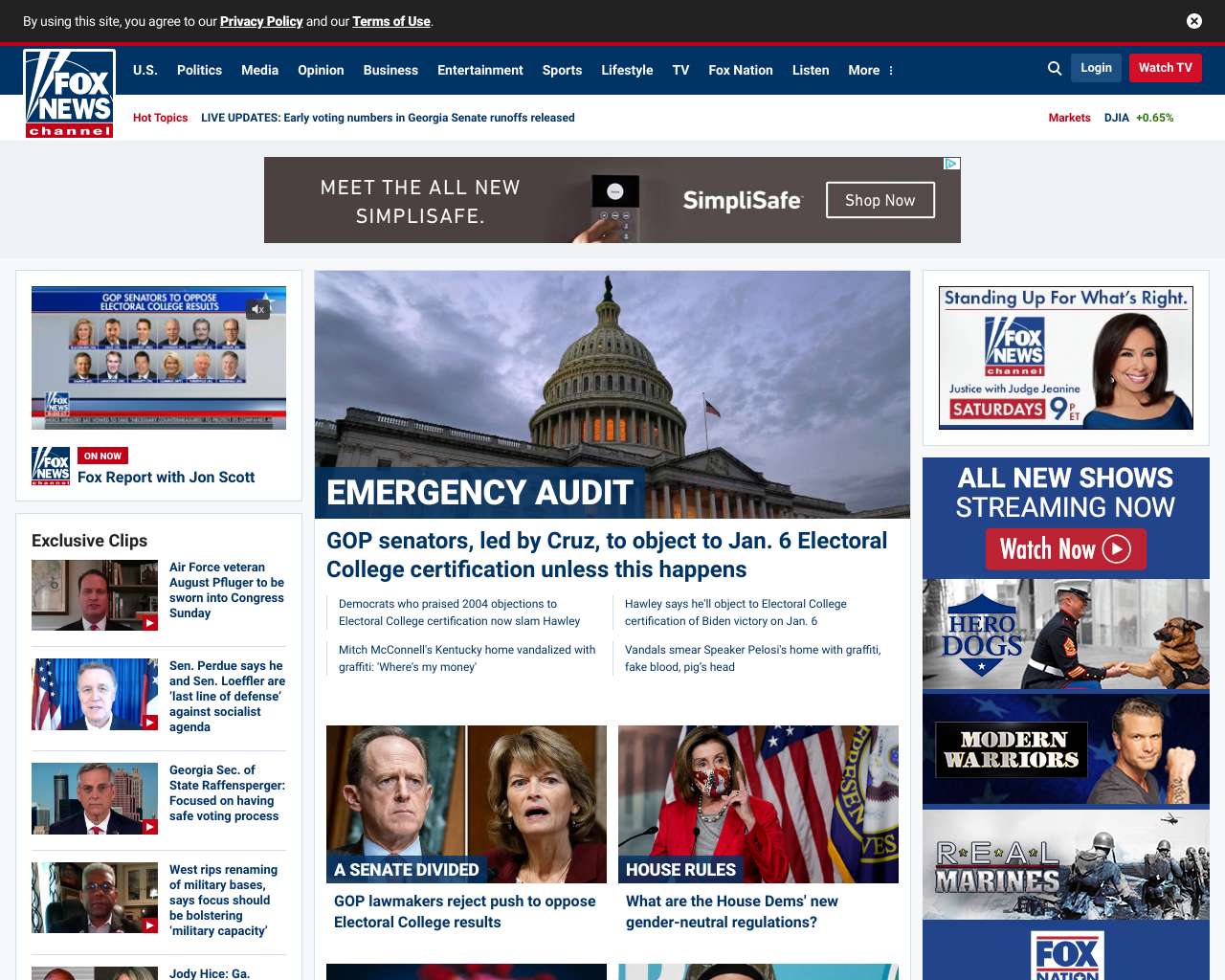This is an image depicting a detailed screenshot of a Fox News website. In the upper left corner, the Fox News logo is prominently displayed, accompanied by the tagline "Fox News Channel." A large ad for SimpliSafe occupies the top of the page, contained in a brown rectangular banner. The ad features a person pressing a button alongside the text "Meet the all-new SimpliSafe," with a "Shop Now" call-to-action.

Below the ad, a notable headline features an image of the Capitol building and addresses an ongoing political issue: "Emergency Audit: GOP Senators Led by Cruz to Object to January 6th Electoral College Certification, Unless This Happens." This headline is immediately followed by an article.

On the left side of the webpage, a section titled "Exclusive Clips" showcases four images of various men. Each image has a red play button, allowing users to watch video clips. Below this section, a caption "A Senate Divided" appears, along with images of a white man and a white woman, likely referring to division within the Senate.

On the right side, an ad for a Fox News program features a female reporter with dark hair. The text promotes the show "Standing Up for What's Right," airing Saturdays at 9 p.m. Eastern Time. Another promotion below highlights "All-New Streaming Shows," prompting users to "Watch Now."

Further down on the right, an advertisement labeled "Hero Dogs" features a Marine alongside a German shepherd. Additional promotions include "Modern Warriors," showing a man with a tattoo staring directly at the camera, and "Real Marines," which is accompanied by a black-and-white photo, seemingly from World War II.

Another prominent headline on the right shows Nancy Pelosi wearing a face mask with the title "House Rules: What Are the House Dems' New Gender-Neutral Regulations?" This is aligned with the ongoing political discourse.

Overall, the webpage is a blend of breaking news articles, video clips, and advertisements, providing an in-depth view of the content and promotions currently featured on the Fox News website.